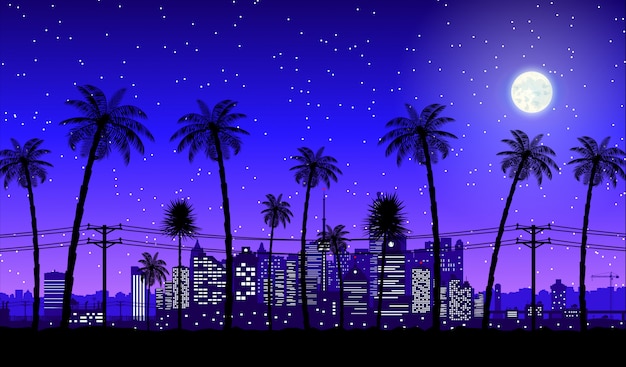This animated scene, set in a rectangular landscape view, vividly portrays a downtown area at night. The dark blue sky, adorned with numerous twinkling white stars, serves as the backdrop, while a radiant full moon glows prominently on the right-hand side. In the foreground, silhouetted black palm trees add a natural element to the urban landscape. In the distance, an array of black skyscrapers rises, their facades dotted with white lights that hint at bustling city life. The sky exhibits a gradient, transitioning from deep blue at the top to a lighter purple near the horizon, suggesting that the sun has recently set.